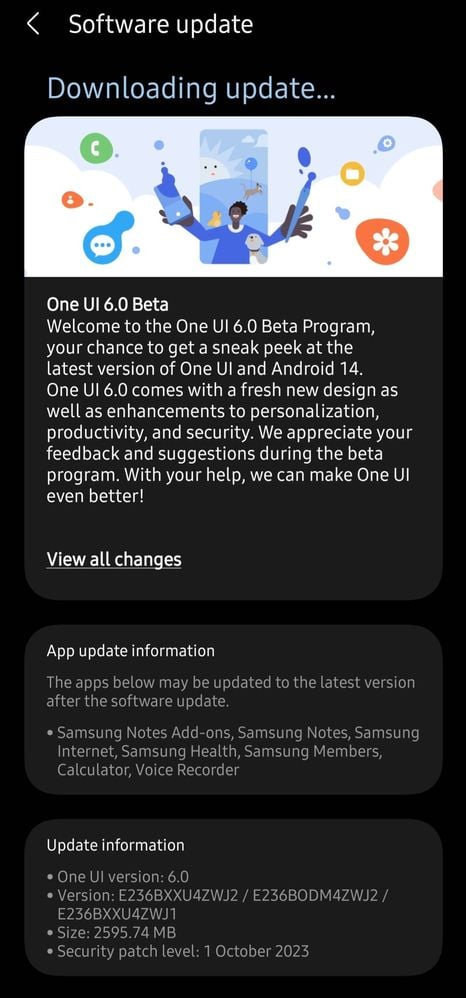A screenshot displaying the download status of a software update for One UI 6.0 Beta on a Samsung device. The screen is in Night Mode with a black background, providing various details about the update process. The text includes specific update information pertinent to Samsung, indicating the update is for either a general phone system or a specific application. The aesthetic of the screen suggests it's an ongoing firmware upgrade on a Samsung smartphone, enhancing both the system's functionality and user experience.